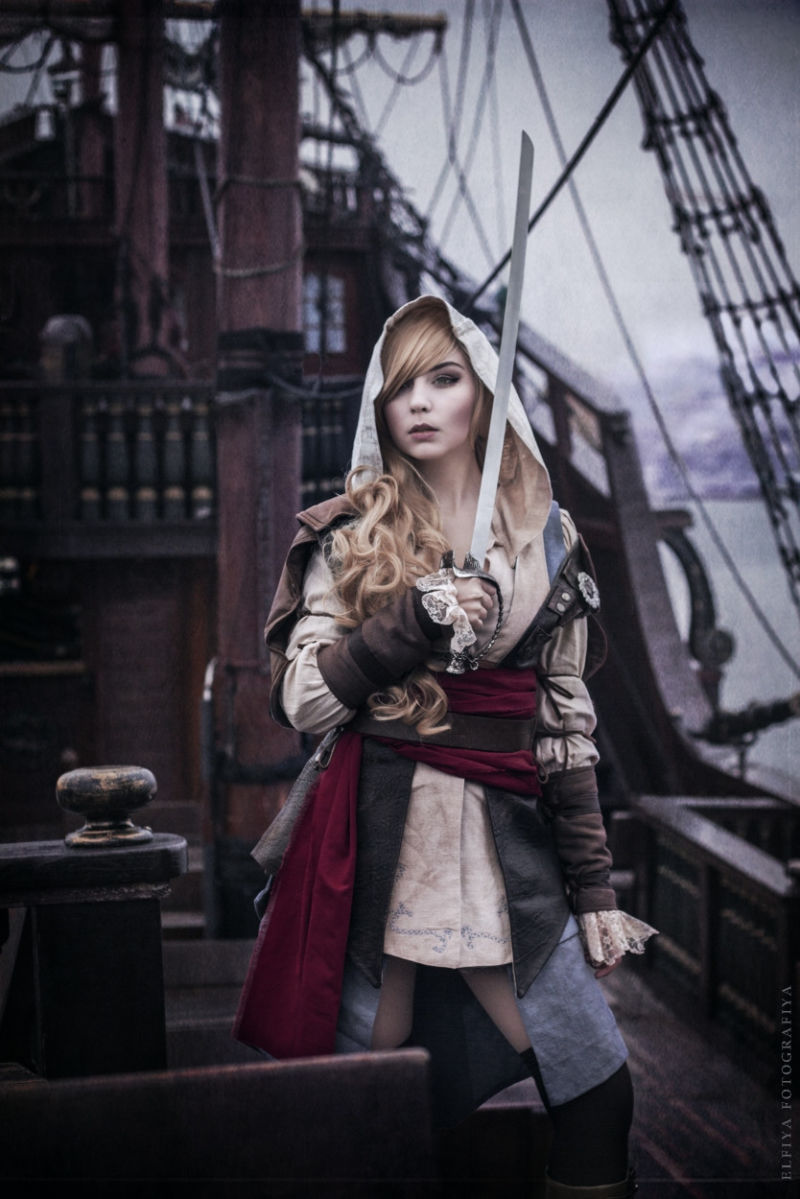This vertically aligned rectangular image features a young woman in her 20s, posing with a sword on an old-timey wooden ship. The background reveals a gray, cloudy sky with thunderclouds forming, adding a dramatic touch to the scene. Positioned just right of center, the woman faces forward, her head slightly turned to the left. She has long, curly blonde hair that cascades over her right shoulder and down past her chest.

She is dressed in a seductive-looking pirate outfit, composed of multiple layers. Her ensemble includes a short-cut, light-colored dress with a dark red sash and a black belt cinched around her waist, adding definition and structure to her attire. Over this, she wears a green vest and long sleeves that end in brown fabric at her wrists. Completing her attire are tall black boots, partially visible below her bare legs, and a matching hood that covers her head, further enhancing her pirate-like appearance.

In her right hand, held in front of her chest, is a sword pointing straight up and slightly to the right, extending above her head. Her left arm rests casually at her side. The ship around her is brown and wooden, with visible sails and a large wooden mast to her left. Further details include wooden columns with brass knobs, the ship's edge to her right, and netting extending from the upper right corner. The scene also captures some distant water and land. In the lower right side of the image, vertical fine print includes the word "photography," though the preceding word remains unclear.